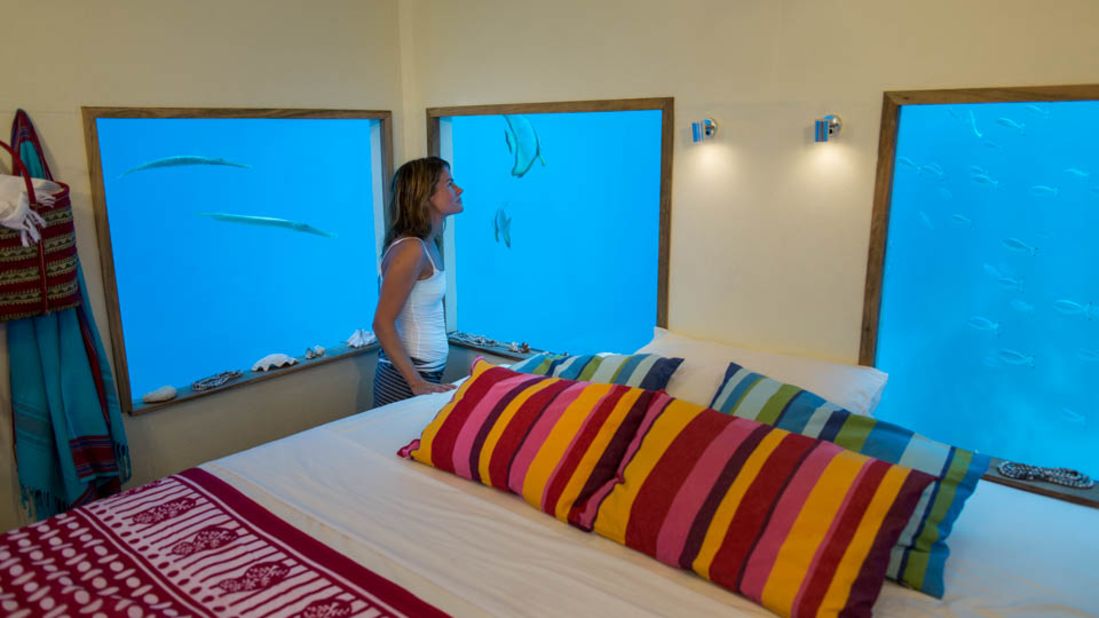In this vividly detailed photograph, a young woman stands in awe in the corner of an underground hotel room, mesmerized by the aquatic view through three large, square windows framed in brown wood. The windows, which provide a stunning underwater perspective with a blue hue, display a variety of marine life including large and small fish. The room's focal point is an oversized bed situated in the center, adorned with crisp white sheets and a red blanket patterned with white stripes and spots. The bed is further decorated with five pillows; the two front pillows showcase pink and orange stripes, the middle two display green and blue stripes, and the backmost pillow is plain white. The girl's attire includes a white tank top with spaghetti straps and a striped skirt, perfectly complementing the serene underwater setting. The room's ambiance is enhanced by two wall-mounted lamps in front of her, casting a warm glow, while her bag and jacket are neatly hung on a coat rack. Shelves lining the window frames add a touch of practicality to this captivating, submerged hideaway.